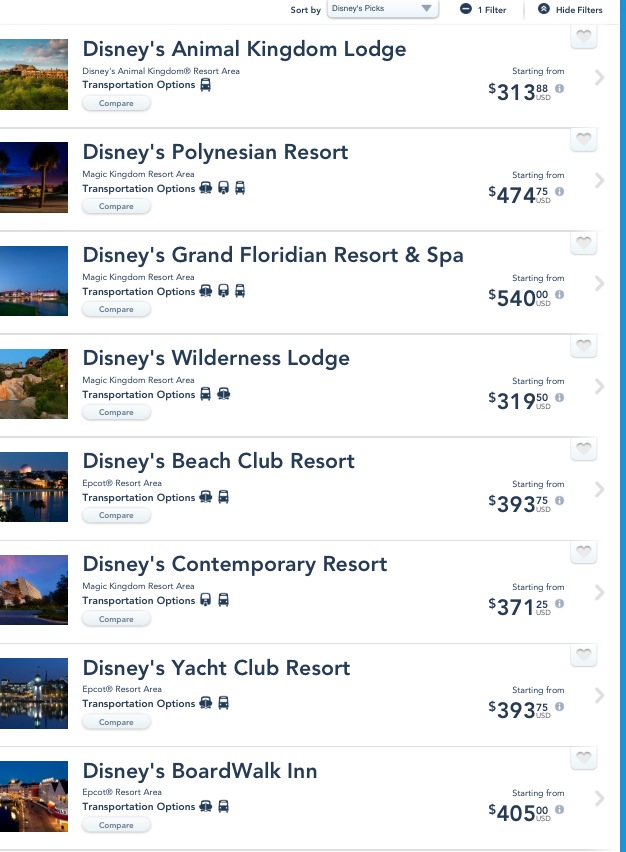**Screenshot Description of Disney Resorts and Inns Pricing**

This screenshot presents a detailed overview of various costs for Disney resorts and inns. At the top of the screen, "Sort by" is displayed in a blue font, accompanied by a dropdown menu labeled "Disney picks." The upper-right corner features options to apply one filter and to hide filters.

The main section lists different categories of Disney accommodations, each showcasing an image of the respective location on the left-hand side. Here are the detailed listings:

1. **Disney's Animal Kingdom Lodge**
   - **Resort Area**: Disney's Animal Kingdom Resort
   - **Transportation Options**: Bus or shuttle
   - **Starting Price**: $313.88 USD

2. **Disney's Polynesian Resort**
   - **Resort Area**: Magic Kingdom Resort Area
   - **Transportation Options**: Boat, trolley, car, or bike/scooter
   - **Starting Price**: $470.00 - $475.00 USD

3. **Disney's Grand Floridian Resort and Spa**
   - **Resort Area**: Magic Kingdom Resort Area
   - **Transportation Options**: Boat, trolley, car
   - **Starting Price**: $540.00 USD

4. **Disney's Wilderness Lodge**
   - **Resort Area**: Magic Kingdom Resort Area
   - **Transportation Options**: Trolley, boat
   - **Starting Price**: $319.50 USD

5. **Disney's Beach Club Resort**
   - **Resort Area**: Epcot Resort Area
   - **Transportation Options**: Boat, trolley
   - **Starting Price**: $393.75 USD

6. **Disney's Contemporary Resort**
   - **Resort Area**: Magic Kingdom Resort Area
   - **Transportation Options**: Trolley, motorbike-like vehicle
   - **Starting Price**: $371.25 USD

7. **Disney's Yacht Club Resort**
   - **Resort Area**: Epcot Resort Area
   - **Transportation Options**: Boat, trolley
   - **Starting Price**: $393.75 USD
   
8. **Disney's Boardwalk Inn**
   - **Resort Area**: Epcot Resort Area
   - **Transportation Options**: Boat, trolley
   - **Starting Price**: $405.00 USD

The descriptions provide insight into the visual and functional elements of each resort, making it easy to compare prices and transportation options.